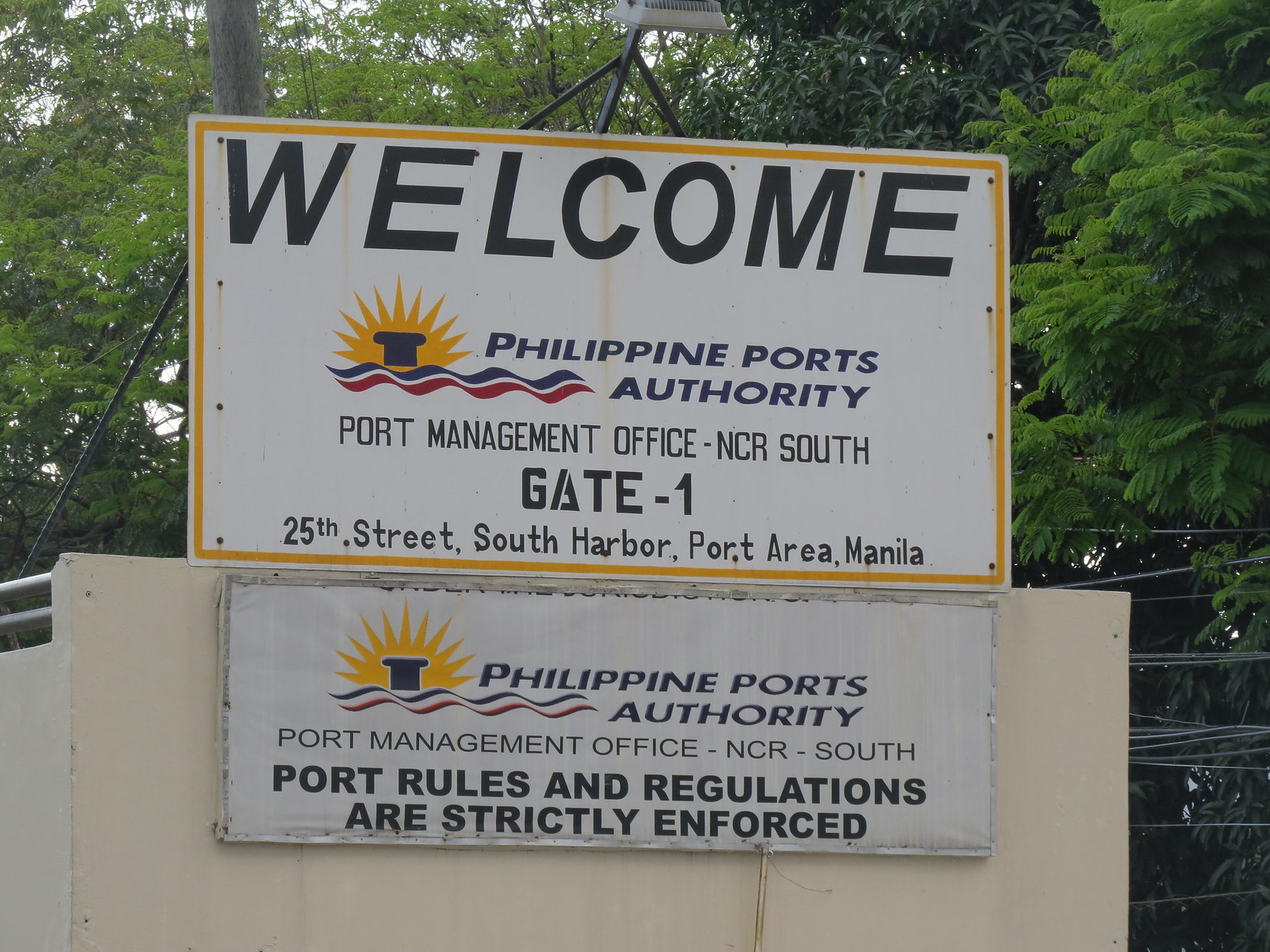This photograph captures a pair of rectangular signs mounted on a white, cream-painted wall, set against an outdoor backdrop featuring lush green trees and visible cable wires attached to light poles. The larger sign on top, outlined in yellow, prominently displays in bold black letters, "Welcome" followed by the "Philippine Ports Authority" with a multicolored logo next to it. Below that, it states "Port Management Office, NCR South, Gate 1, 25th Street, South Harbor, Port Area, Manila." The smaller sign beneath reiterates "Philippine Ports Authority" and "Port Management Office, NCR South," and emphasizes in darker black letters, "Port Rules and Regulations are Strictly Enforced." The signs are accented by an attached light, indicating that the photograph was taken during the daytime. To the left, a segment of iron railing is visible, adding to the scene's infrastructural details.